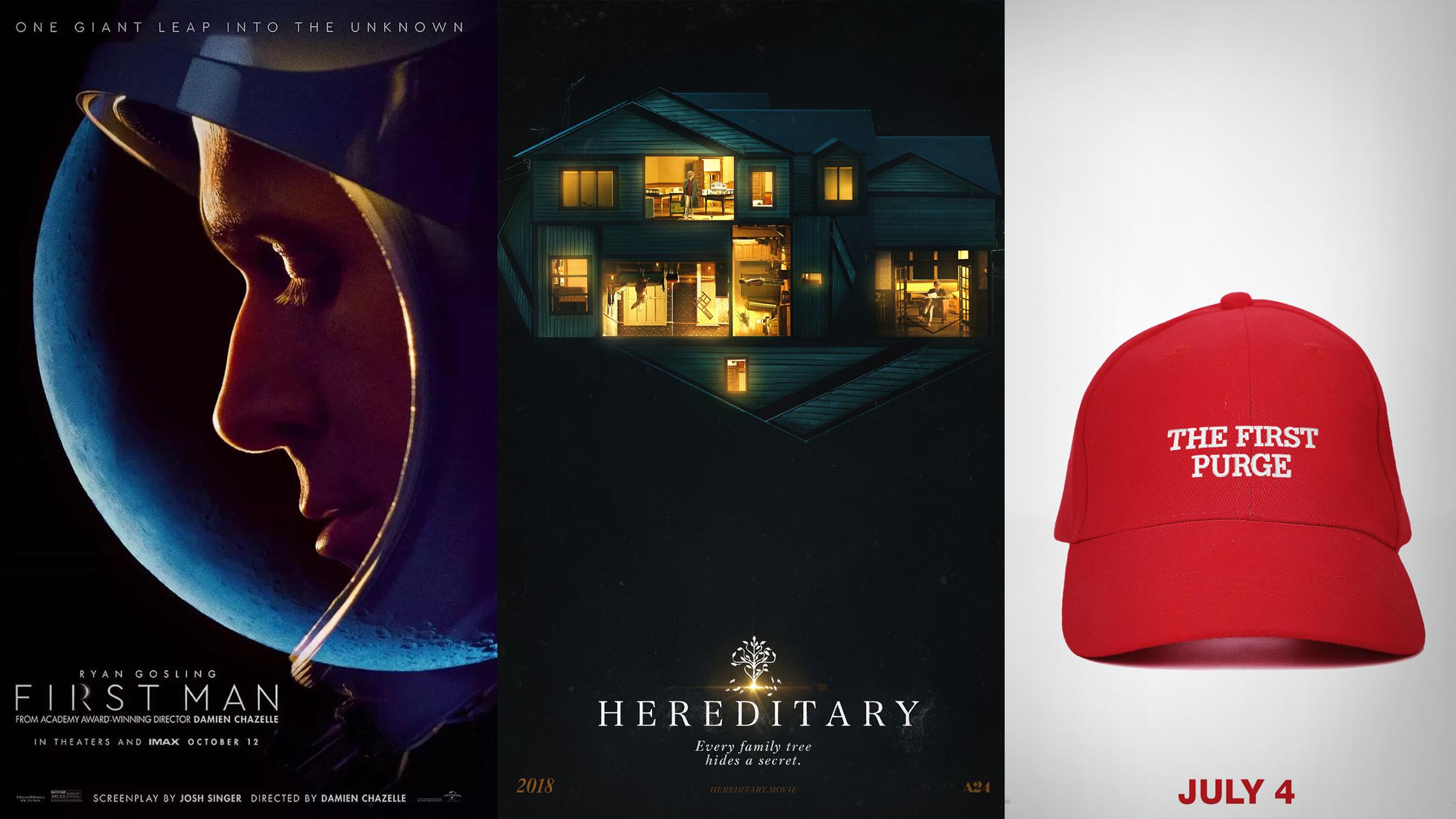The image is a montage of three distinct movie posters displayed side-by-side. The first poster, against a black background, features a blue and black moon with a man's profile integrated into it. Above this imagery, in bold white text, it reads "One giant leap into the unknown." In the lower left-hand corner, it states "Ryan Gosling, First Man," and at the bottom of the poster, additional white text credits the screenplay by Josh Singer and direction by Damien Chazelle, with a release date of "In theaters and IMAX October 12th." The second poster showcases a dimly lit two-story house at night, possibly by a body of water, with all its lights on and windows open. Centered at the bottom, it says "Hereditary" with the tagline "Every family tree hides a secret," and in the lower left-hand corner, it mentions the release year, "2018." The third poster presents a striking contrast with a white background and a red baseball cap prominently displayed in the center. On the cap, in bold white letters, it reads "The First Purge," and below it, in red letters, it indicates the release date, "July 4th."